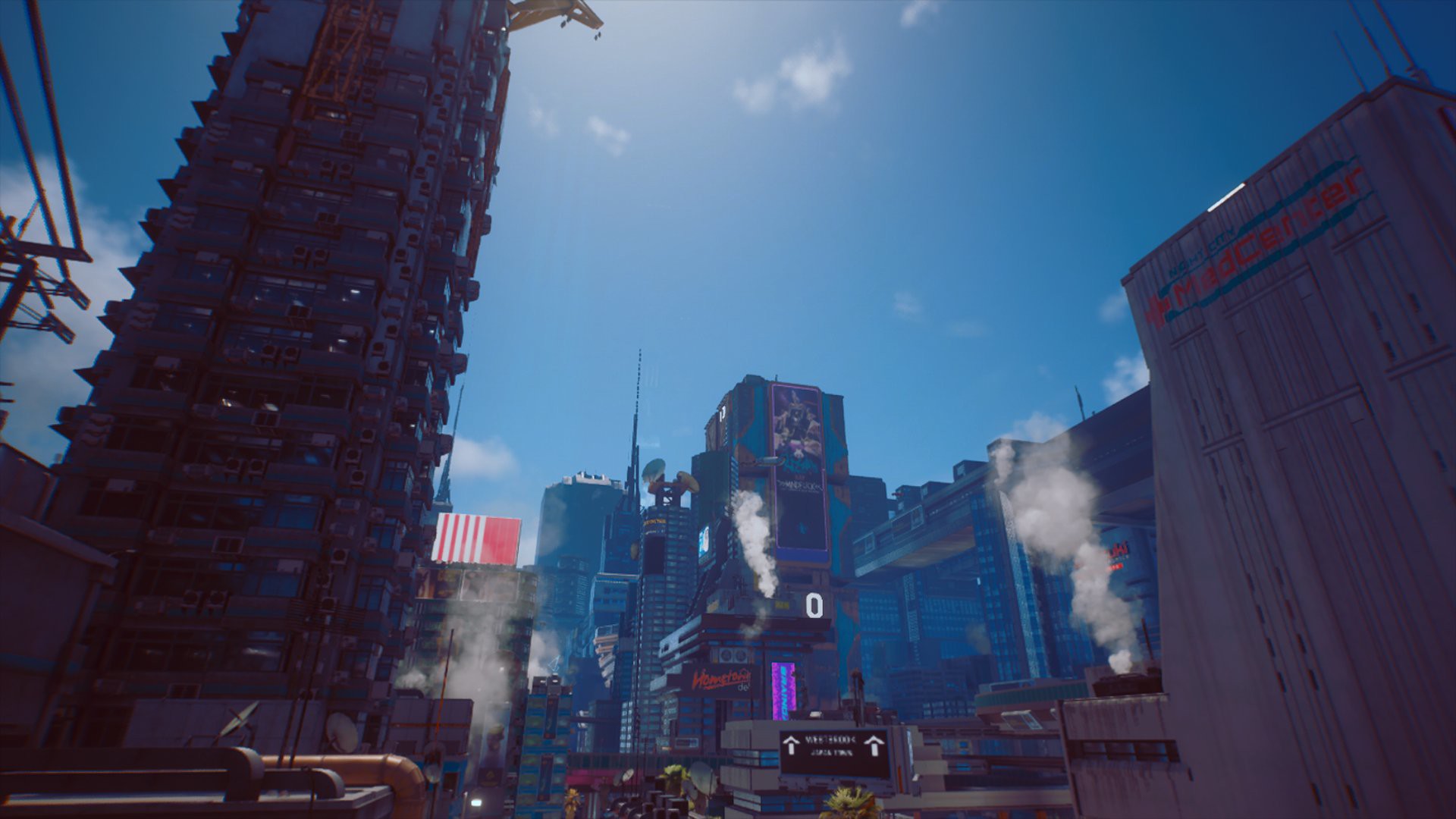This image appears to be a computer-generated night scene of a city, presenting a surreal juxtaposition of elements that blend both day and night characteristics. The sky is an unrealistically bright medium blue, punctuated with white puffy clouds that give it a daytime appearance. Contrastingly, the city's buildings beneath exhibit darker hues that imply this is at least dusk, if not a night scene.

In the center of the image, several buildings, which seem slightly more distant, are colored in medium to dark bluish-gray tones. The tallest among these structures stands at about three or four stories high. Below, there's a prominent sign featuring red writing, though the text is not discernible. A large building in this area has a patio extending outward, accompanied by what seems to be a street sign on its side.

To the right, a substantial gray building displays some red text that is also unreadable. From at least three points on this building, white smoke billows upward, enhancing the atmospheric complexity. Adjacent to this, a towering structure that resembles a parking garage, possibly 15 floors high, is present, albeit its purpose is ambiguous, potentially indicating a building under construction with numerous open areas.

Adding to the scene's eclectic nature is a flag positioned near this tall structure. The flag is distinctly half red with vertical red stripes on a white background, contributing further to the image's blend of vibrant and muted tones.